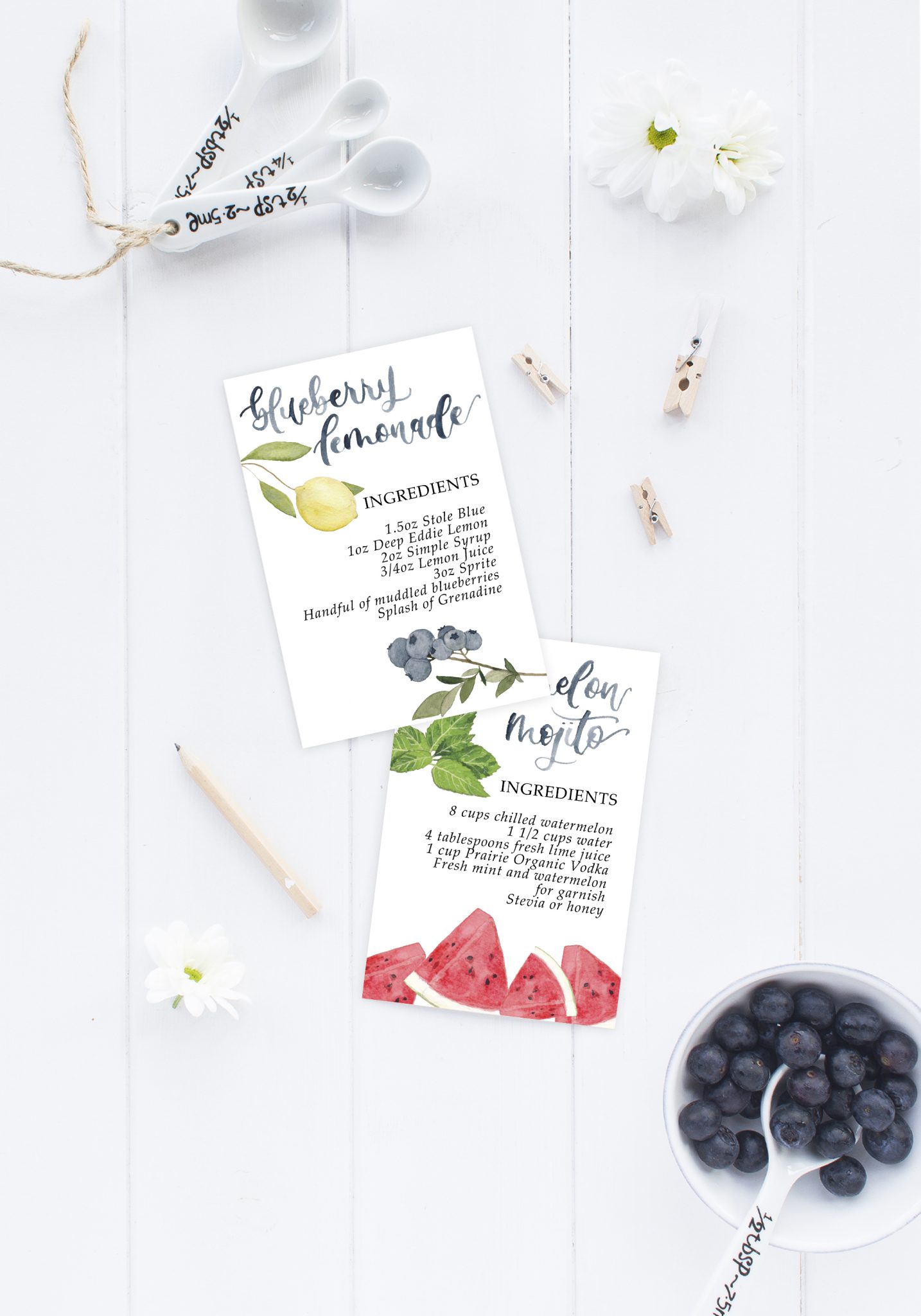The image showcases a meticulously arranged white wooden table with vertical lines, creating a clean and organized aesthetic. In the top left corner, tied together with twine, are three white measuring spoons labeled as half teaspoon, quarter teaspoon, and half tablespoon. Adjacent to the spoons are two white flowers with green stems. Below them, there are three light beige clothespins, with one being half beige, half white. 

Central to the image are two well-detailed recipe cards. The first card on the left is for a **Blueberry Lemonade**, garnished with images of lemons and blueberries. The ingredients listed are:
- 1.5 oz Stolichnaya Blue
- 1 oz Deep Eddy Lemon 
- 2 oz simple syrup
- 3 oz lemon juice
- 3 oz Sprite
- A handful of muddled blueberries
- A splash of grenadine

Next to it, the second card is for a **Melon Mojito**, displaying slices of red watermelon and mint leaves for garnish. Its ingredients include:
- 8 cups chilled watermelon
- 1.5 cups water
- 4 tbsp lime juice
- 1 cup Prairie Organic Vodka
- Fresh mint and watermelon for garnish
- Stevia or honey to taste

To the left of these cards, a pencil lies perfectly parallel to them. Below the melon mojito recipe, there's another white flower similar to the top ones. On the bottom right, a small white bowl filled with blueberries is situated, with a white half-tablespoon measuring spoon lying inside. This artful arrangement not only highlights the refreshing nature of these summer drinks but also brings out the beauty in everyday kitchen tools and ingredients.